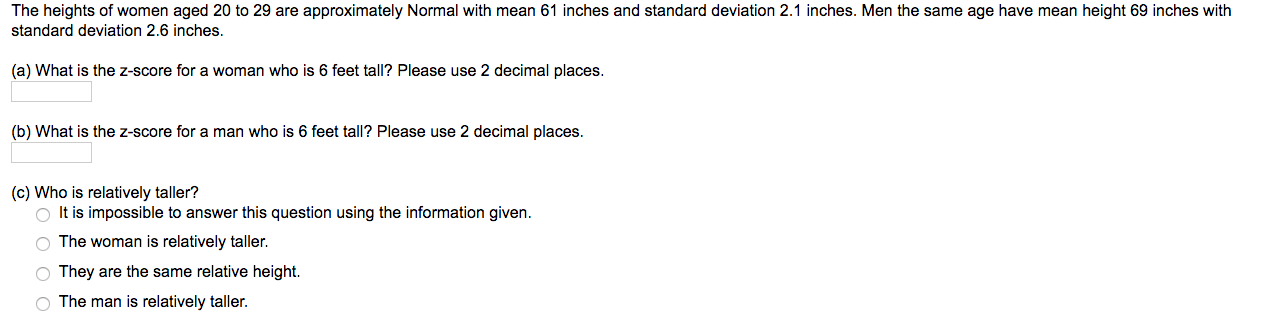In this image, we see a screenshot from a document or a website with a white background and black text. The text appears to be describing a math problem related to heights of individuals. Specifically, it states that the heights of women aged 20 to 29 are normally distributed with a mean of 61 inches and a standard deviation of 2.1 inches. Men of the same age have a mean height of 69 inches with a standard deviation of 2.6 inches.

Following this information, there is a section labeled "Part A" with a question asking for the Z score of a woman who is 6 feet (72 inches) tall, instructing the answer to be provided to two decimal places. Below this question is a rectangular answer box where responses can be entered.

Next, "Part B" asks for the Z score of a man who is 6 feet (72 inches) tall, also requiring the answer to be given to two decimal places, accompanied by another answer box.

Finally, "Part C" poses a multiple-choice question asking who is relatively taller: the woman, the man, or if it is impossible to determine from the given information. The options provided are:
- It is impossible to answer this question using the information given.
- The woman is relatively taller.
- They are the same relative height.
- The man is relatively taller.

Each option has a corresponding bubble to select an answer. Notably, the initial line of text explaining the math question extends almost twice as far across the page as the following questions and answer boxes.